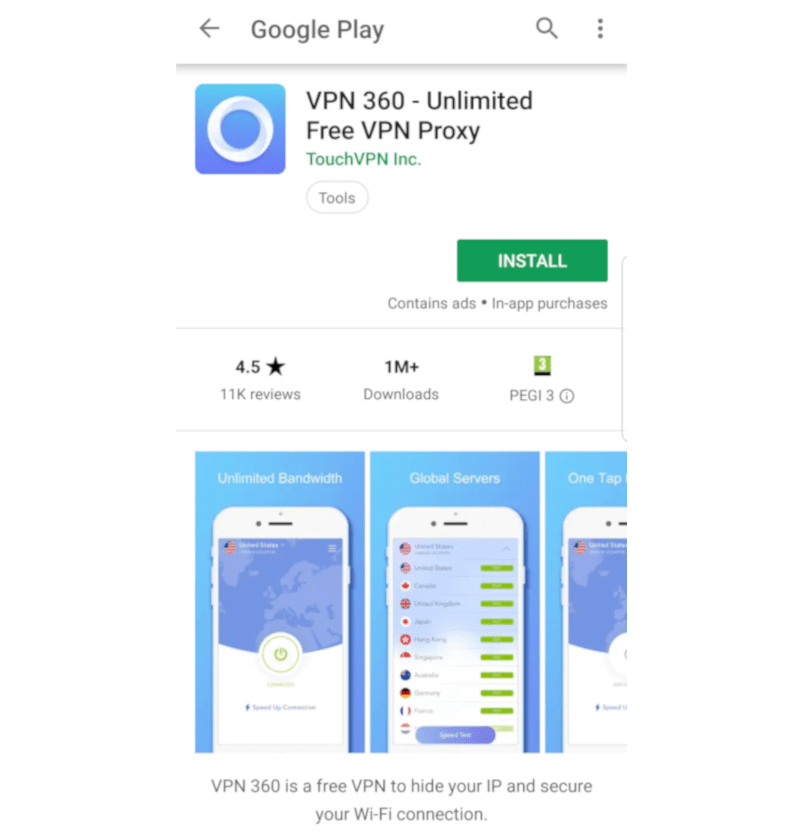The vertical rectangular image showcases a web page from the Google Play Store featuring the VPN app "VPN 360 - Unlimited Free VPN Proxy". At the top, the screen displays the standard Google Play header in gray text with a back arrow on the left, followed by a search icon on the right. Below this, a medium gray banner spans the width of the page. 

Prominently centered below the banner is the app’s name, "VPN 360 - Unlimited Free VPN Proxy," in bold black text. Just below, the developer name "TouchVPN Incorporated" is written in green text. On the left side, the VPN 360 logo features a bright blue square with rounded corners, containing a white circle with subtle light gray shadowing in the center.

Underneath the app name and logo, a white button with a gray border reads "Tools" in gray text. To the lower right, a dark green button labeled "Install" in white capital letters invites you to download the app. Small gray text beneath the button indicates that the app contains ads and in-app purchases.

Further down, the image shows a star rating of 4.5 based on 11,000 reviews, along with over 1 million downloads. The PEGI 3 rating is displayed, with the number '3' inside a green box.

The bottom portion of the image features several vertical rectangular sections with blue backgrounds. These sections display smartphone images emphasizing the key features of the VPN app, including unlimited bandwidth, multiple servers, and quick one-tap connectivity, although the last word is partially cut off.